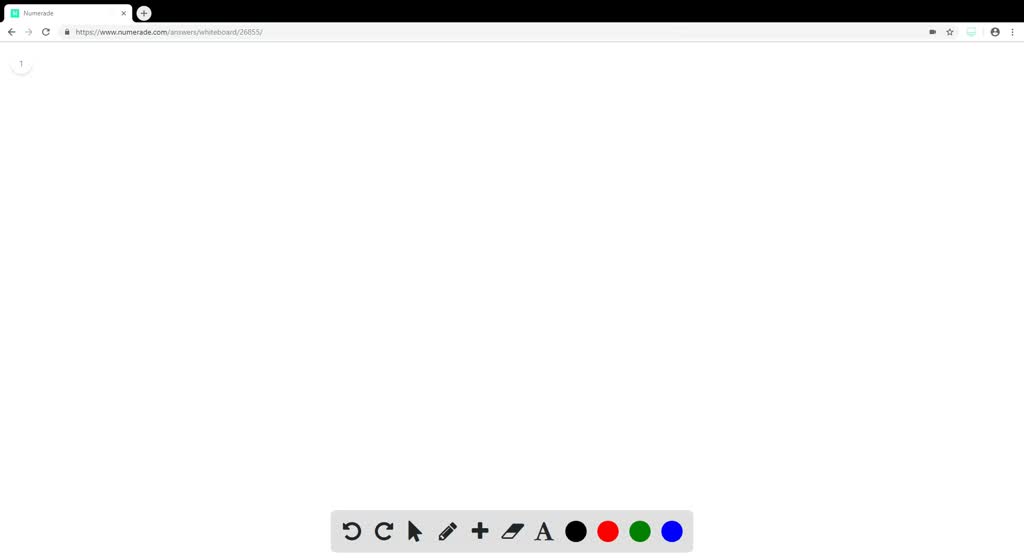This image is a landscape-oriented screenshot taken from a PC, predominantly featuring a plain white background. At the top of the screenshot, a black bar runs horizontally across the screen, anchoring various elements of the interface. In the top left corner of this bar is a white tab with a square green icon beside an indiscernible tab name due to its blurriness. 

Directly below this is the URL bar, also white, containing a website address that is too small to read. To the left of the URL bar are navigation icons: a black refresh icon, a grey forward icon, and a black back icon. On the right side of the URL bar are various symbols, including a favorites icon represented by a star with a white interior and a black border, and a profile icon depicted as a black circle with a white silhouette of a head and shoulders inside it.

The rest of the screenshot is completely blank, save for a grey rectangular menu bar positioned centrally at the bottom of the image. This bar is dedicated to editing and drawing tools and displays several icons in black. From left to right, these include an undo button with a counter-clockwise arrow, a redo button with a clockwise arrow, a mouse icon, a pen icon, a plus icon, an eraser icon, and an 'A' icon indicating a textbox. Additionally, there are four circles in plain colors: black, red, green, and blue, likely representing different color options for drawing or editing.